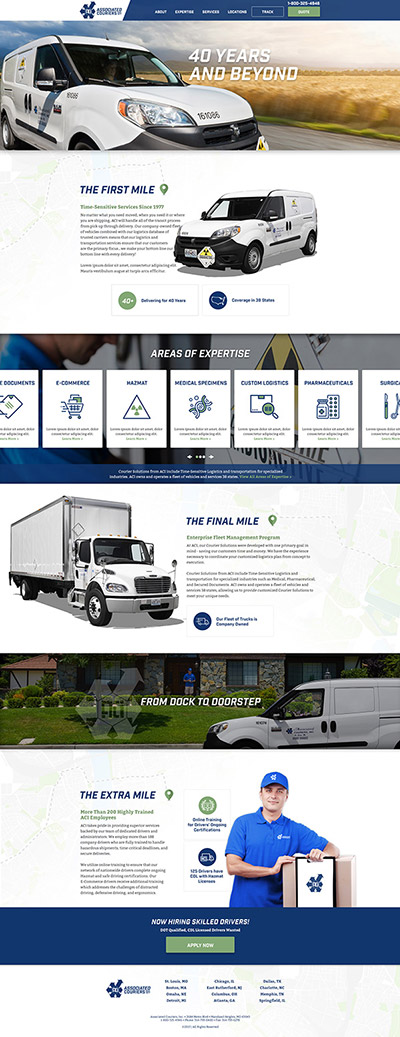The image depicts a poorly designed website advertisement, ostensibly for Progressive Insurance, though the actual identity is unclear due to illegible text. The top third of the ad features a predominantly white background with an indistinguishably small logo and company name. Navigation options such as "Home" and various offerings are spread across the header, but none stand out due to their diminutive size.

A prominent green button, labeled "40 years and beyond," is visible. Below this, a clean white van is shown driving forward. While the front license number is legible, crucial branding or contact details on the vehicle's side are obscured or too small to decipher. The ad mentions "The First Mile," accompanied by a symbol and an unreadable paragraph.

Further down, the ad introduces a green and a blue logo, again with text too small to be practical. Subheadings like "Areas of Expertise," listing capabilities such as e-commerce, appear but with little context. Conclusively, the bottom of the ad references "The Final Mile," still leaving the viewer guessing about the company's identity or services, presumably related to travel or shipping. Overall, the advertisement suffers from poor legibility and ineffective communication.